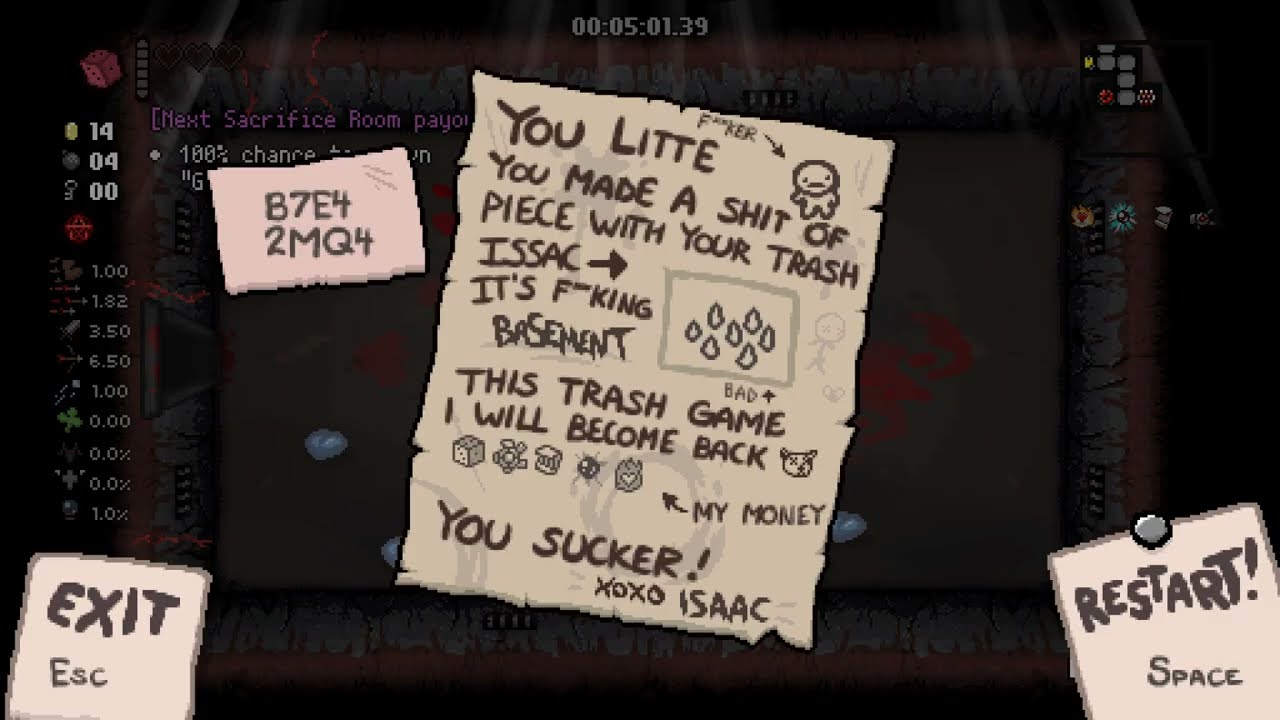The image depicts a dark digital screen that resembles the start of a game on a cell phone or computer. The background is pitch black, and various digital notes and illustrations appear to be tacked onto it. On the lower left corner, there's a beige square labeled "exit" with smaller text "ESC," above which is a pinkish rectangle displaying a code "B7E4 2MQ4." Meanwhile, the lower right corner features another beige rectangle with "RESTART!" and "Space" in handwritten text, seemingly held by an illustration of a tack.

Dominating the central part of the screen is a large, dirty-white, torn piece of paper with black writing and various drawings. The message, laden with foul language, reads, "You little, ULITTE, you made a shit of piece with your trash, Isaac. It's fucking basement, this trash game. I will come back, you sucker." The note is punctuated with hand-drawn icons and annotations such as "My money," some figures like dice, gear, sandwich, bug, and a smiling face. The note concludes with "XOXO, Isaac." Above the chaotic notes, there's a counter displaying "50050139," which suggests a countdown or some form of scoring mechanism, solidifying the impression that this scene is from within a game environment.